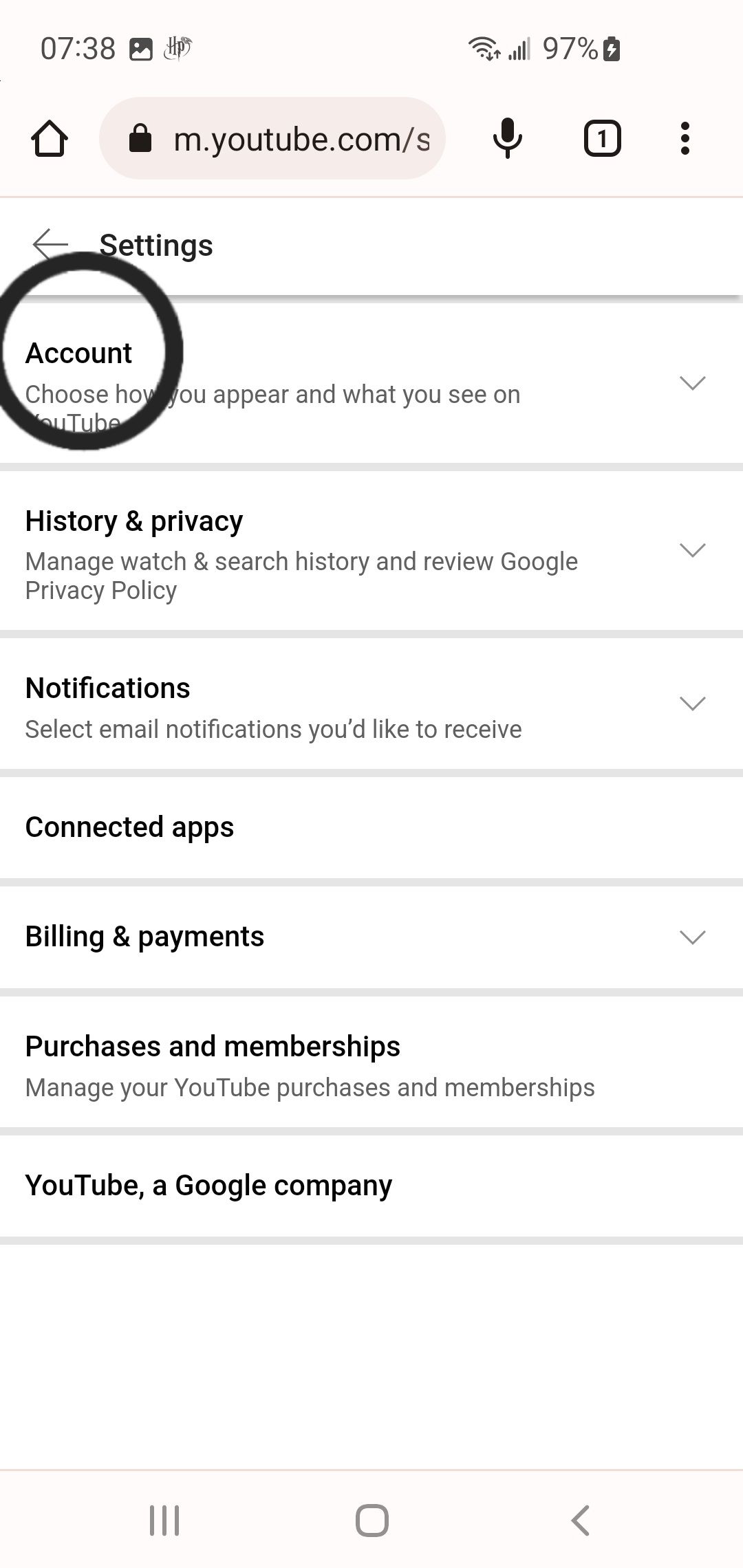**Detailed Caption:**

The image is a screenshot of a smartphone showing how to access YouTube's account settings. The phone has a battery level of 97% and displays the time as 7:38. It is unclear whether the device is an Android or an iPhone. The URL bar contains the text "m.youtube.com/s" but is partially cut off. To the right of the URL bar, there is a microphone icon and an indicator showing one tab is open, followed by three vertical dots, which likely represent more options.

Below the URL, the screenshot displays a section from the YouTube mobile website titled "Settings." This section allows the user to navigate through various setting options. At the very top, "Account" is highlighted and encircled in a large black circle with the subtitle, "Choose how you appear and what you see on YouTube." 

Following "Account," there are six more sections, each divided by a thin line or "div":
1. **History and Privacy** - Manage watch and search history and review Google's privacy policy.
2. **Notifications** - Select email notifications you'd like to receive.
3. **Connected Apps** - Manage applications connected to your YouTube account.
4. **Billing and Payments** - Information about bill payments, purchases, and memberships.
5. **YouTube** - Identifying YouTube as a Google company.

At the very bottom of the image, you can see the smartphone's navigation buttons.